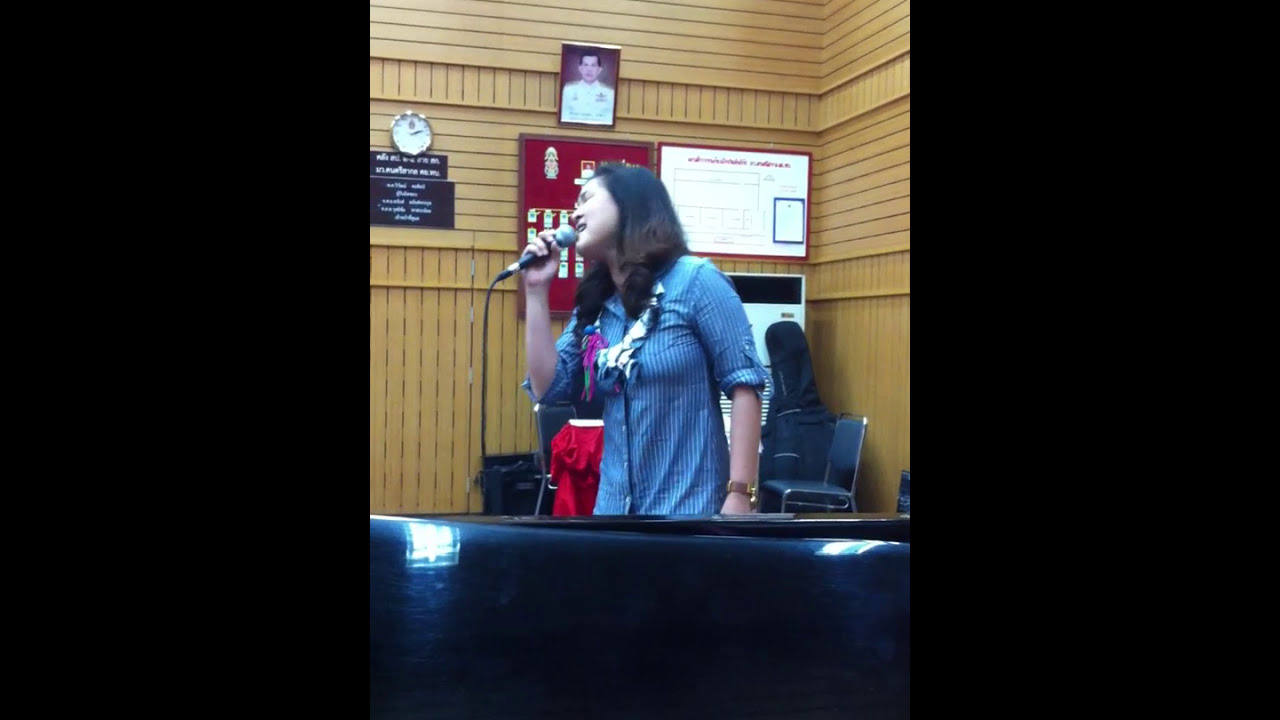In the center of this color photograph, a young woman aged about 20 to 25 years old is passionately singing into a microphone she holds in her right hand. She faces towards the left, showcasing her shoulder-length, dark brown hair and glasses. She is dressed in a buttoned-up blue striped shirt with the sleeves rolled up to her elbows, featuring vertical stripes in varying shades of blue. Draped around her neck is a colorful scarf. The setting appears to be an indoor auditorium, likely during a live performance. Behind her, a chair occupies the corner of the room in front of a back wall adorned with various framed items, which may include certificates or awards. Above these is a picture of a dark-haired Asian man in a white dress uniform. To the top left of the image is a rounded item, possibly a clock, with some signs underneath. The walls exhibit a mix of horizontal hardwood planks and vertical blank sections. The entire photograph is in portrait orientation and is inset within a black landscape-oriented background, adding a frame-like border that accentuates the scene. Colors spotted in the image include shades of blue, black, gray, red, purple, green, silver, tan, and gold. The overall ambiance suggests a midday indoor setting, perhaps in front of a crowd or during a public event.